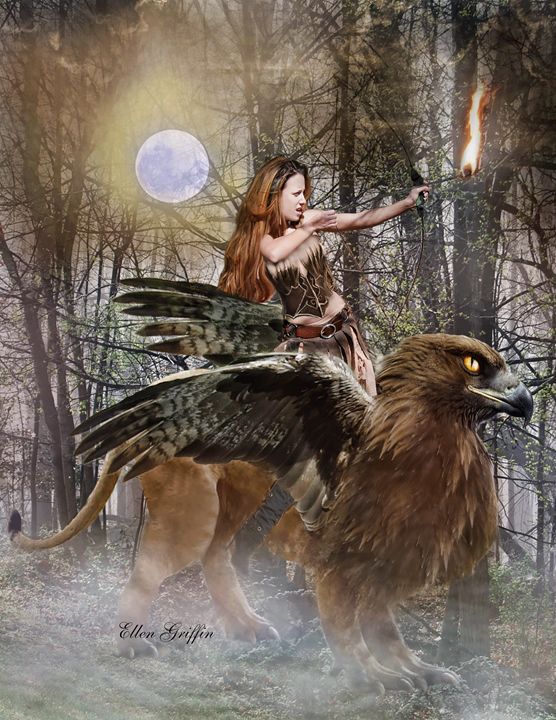The image depicts a detailed digital artwork by Ellen Griffin, as indicated by the signature at the bottom. Set in a foggy, nighttime woodland with numerous bare trees and a mossy forest floor, the scene is illuminated by a full moon positioned unrealistically in front of the tree branches. Central to the composition is a mythical griffin, featuring the face of a hawk with a curved beak, amber eyes, and large black-tipped wings, while its body and tail resemble those of a lion. A barbaric-looking woman with long reddish-brown hair, fair skin, and wearing rustic clothing made of animal materials—complete with boots, a belt, and a half-shirt—sits astride this griffin. She is intensely focused, pulling back a bow to release a flaming arrow. The griffin's detailed plumage and the woman's determined posture contribute to the dynamic and fantastical aura of the artwork.